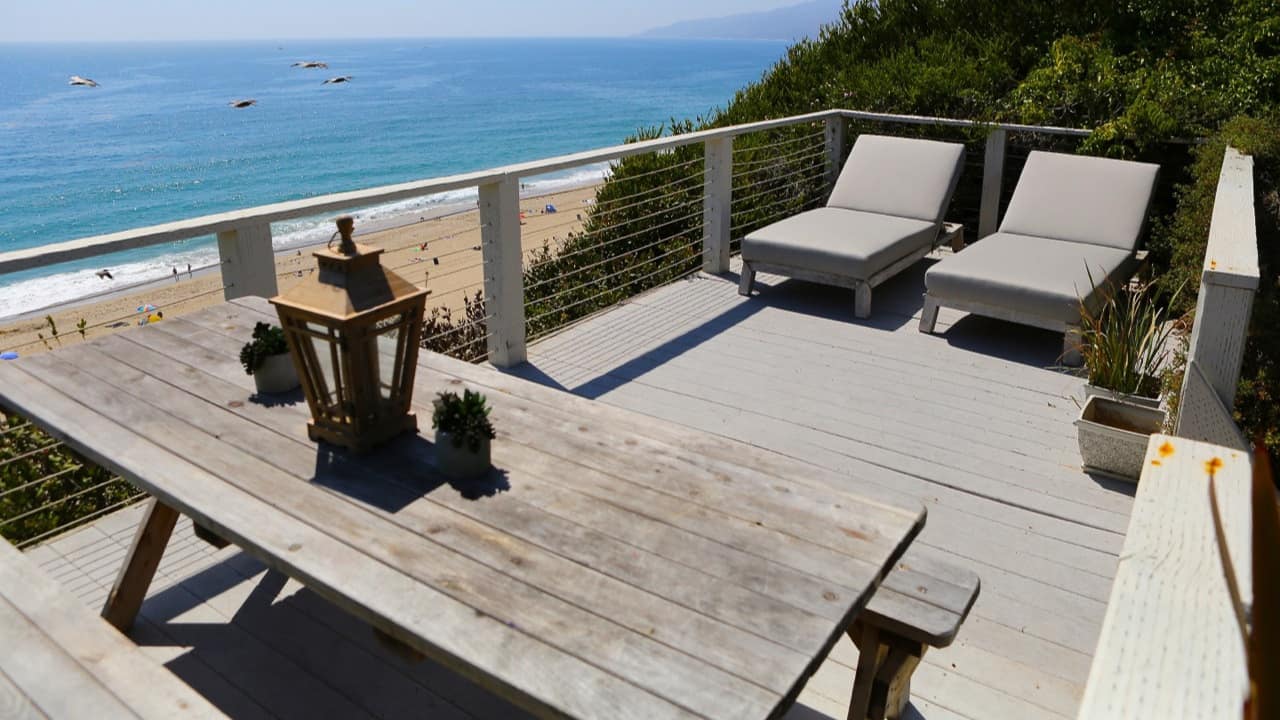The image captures a picturesque deck overlooking a serene beachside setting. On the top left, the vast, light blue ocean spans across the frame, with intriguing figures that resemble whales breaching the water, adding an almost surreal touch to the scene. The water's texture appears slightly altered, hinting at possible digital enhancement. 

In the midground, a strip of golden sand is dotted with tiny, indistinct figures of beachgoers, too far to discern specific details about their attire. At the heart of the photograph, the deck commands attention with its simplistic charm. 

Towards the back of the deck, lush bushes provide a vibrant green backdrop, complementing the two silver-gray reclining lawn chairs positioned side by side. A modest planter rests beside them, adding a touch of nature to the setup. The deck itself, a weathered wooden structure painted in a soft gray, features sturdy railings composed of silver-gray posts and barrier wires, ensuring safety without obstructing the view.

In the bottom left corner, a rustic picnic table garnished with a couple of small plants and a lantern suggests a cozy spot for evening gatherings. The table, aged and wooden with specks of gray, speaks to years of exposure to the elements, further enhancing the deck’s inviting, lived-in feel.